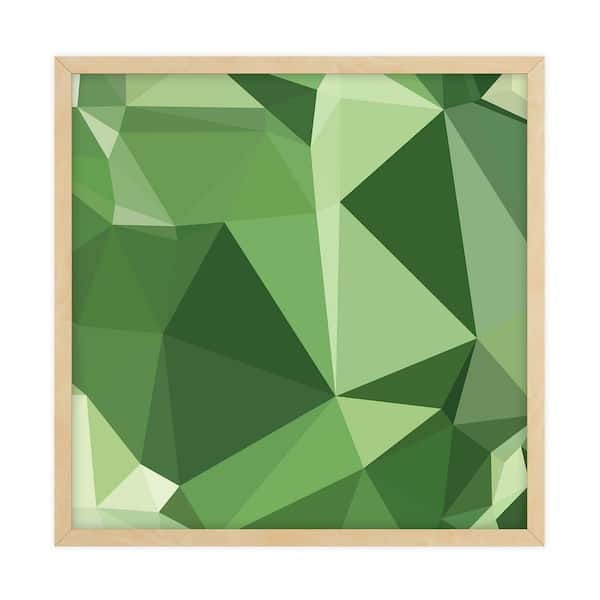The image showcases a piece of conceptual artwork framed in light brown wood. The artwork features an intricate geometric design, composed entirely of various shades of green—ranging from forest green to lime green to olive green. The composition consists of numerous triangle shapes that collectively form a larger, abstract shape, resembling a multifaceted gem with peaks and valleys, giving a sense of depth and three-dimensionality. The artwork is devoid of any text, ensuring the viewer's focus remains on the dynamic interplay of the green triangles. The frame and the artwork itself stand out clearly against a plain background, highlighting the detailed and imaginative design.